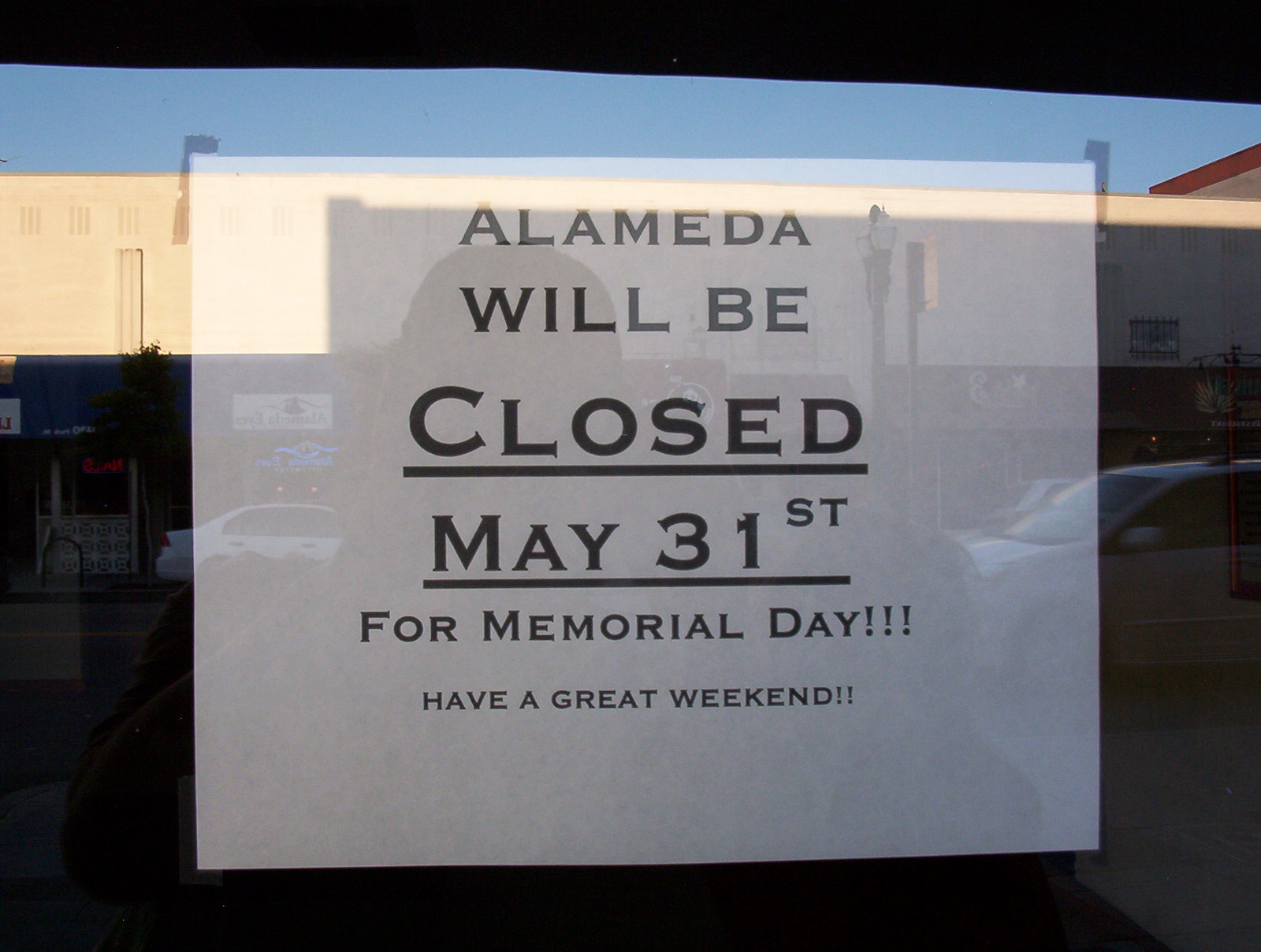The image displays a white piece of paper taped to the inside window of a business, prominently stating: "Alameda will be closed May 31st for Memorial Day," with "closed" and "May 31st" in a larger, bold, and underlined font. The sign also wishes: "Have a great weekend," punctuated by multiple exclamation points. Reflections in the window vividly capture the scene outside: a clear, sunny blue sky, several parked and moving cars, and buildings across the street, indicating other businesses. The faint silhouette of the person taking the picture is also visible in the glass. The sign itself is centered in the window amidst this reflective backdrop. The colors in the scene include whites, blacks, reds, dark orange, beige, and various shades of blue, accentuating the sunny day.